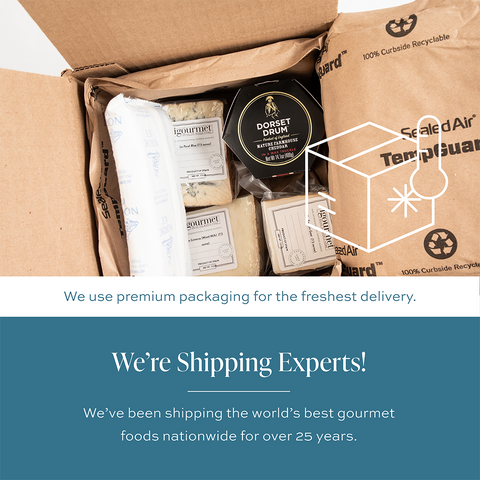The advertisement showcases a detailed photograph of an open corrugated cardboard shipping box, lined with recyclable Sealed Air TempGuard packaging that resembles paper-based air pillows. Inside the box, there are various perishable gourmet items ready for shipment, including what appears to be blue cheese, other cheese varieties, and a jar labeled Dorset Drum, with an ice pack situated on top to keep the contents cold. The photograph is overlaid with an icon featuring an ice cube and a thermometer, signifying temperature control to ensure freshness. At the bottom of the image, a large blue text box declares in bold white font, "We're shipping experts! We've been shipping the world's best gourmet foods nationwide for over 25 years." Above this, another blue font message reads, "We use premium packaging for the freshest delivery," emphasizing the high-quality, protective nature of the packaging.